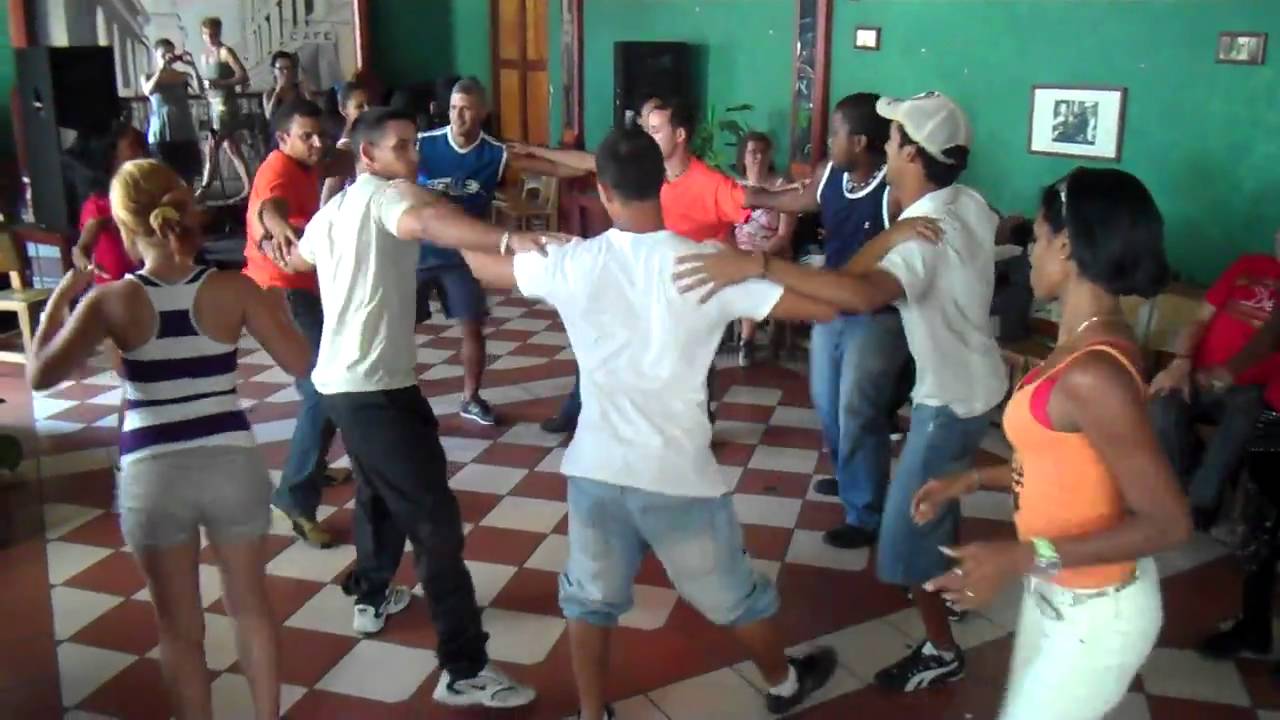The image captures a lively scene inside a room where a group of seven men of diverse races are engaged in a celebratory dance, standing in a circle with their arms linked around each other's shoulders. They are dancing on a tiled floor arranged in a diagonal checkerboard pattern with brown and white squares. In the background, a dark green wall frames the scene, adding contrast to the vibrant activity in the foreground. Among the onlookers, a woman wearing a yellow and orange tank top paired with white pants and a wristwatch on her left hand stands out, attentively watching the dance. Another female observer, dressed in khaki shorts and a purple and white striped tank top, has her back turned to the camera. An intriguing detail is a mirror on the left side of the photograph, partially reflecting the festive moment. The overall ambiance suggests a dance class or a joyous gathering.